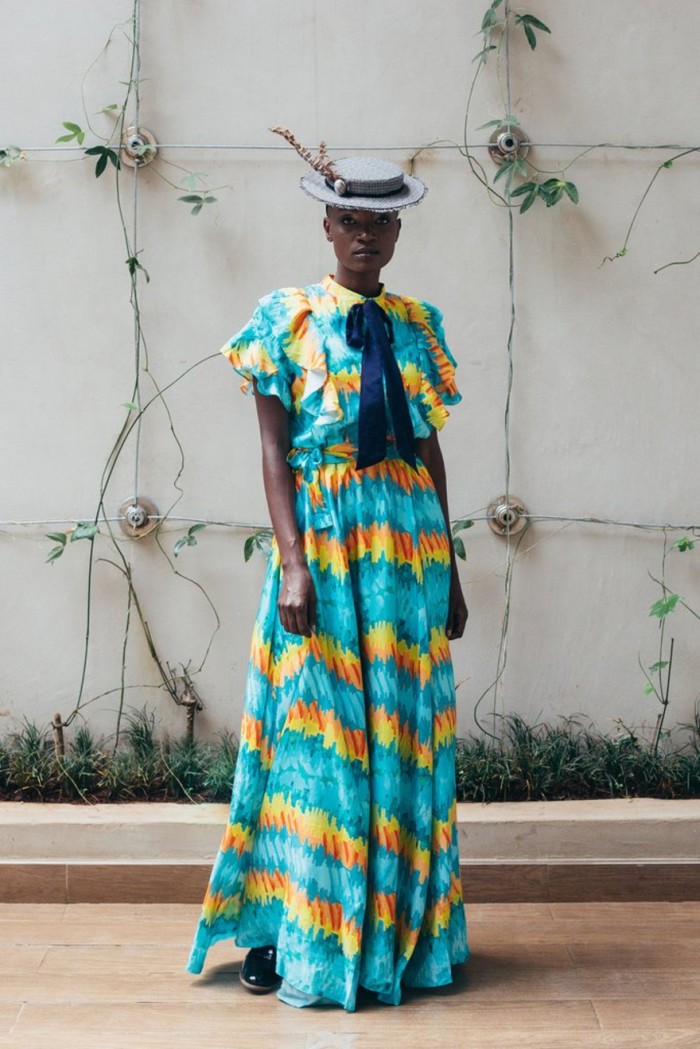In this photograph, an African American female model is standing on a wooden floor, likely inside or on a wooden plank sidewalk. She wears a long, vibrant sundress that predominates with turquoise and features striking bands of yellow and orange stripes, six or seven in total, including one around her waist where a bright turquoise tie strap accentuates her figure. She pairs the dress with a royal blue bow tie with long, hanging parts, adding a contrasting touch of elegance. Her head is adorned with a small mini top hat, which is gray with a flat rim and top. A little brass medallion circles the hat band, and a sprig of plant or a feather adds an organic flair to her ensemble. She sports very short hair and a shiny black shoe peeks from under her dress.

The wall behind her is a beige stucco background with horizontal wires running across, seemingly designed to support vine growth. A few vines and leaves are visible, adding a touch of green to the scene. The wires are supported by metal objects affixed to the wall. Additionally, there's a small ledge with a planter containing grass, complementing the natural theme of the setting. The model gazes directly at the camera with a neutral expression, presenting an image that combines vivid fashion with a subtle botanical backdrop.